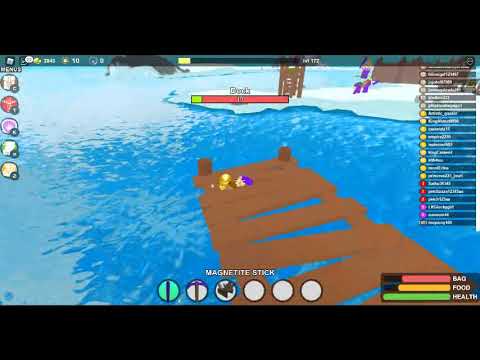The image is a wide rectangular screenshot from a video game, bordered at the top and bottom by thick black strips. The main scene depicts a bright blue body of water that gradually lightens toward the left and top of the image. On the top right, there's a snow-covered white landmass. Extending from the bottom right into the middle is a brown wooden pier with noticeable gaps between the planks, creating a somewhat triangular view of the water below. The water itself appears highly reflective. 

A list of approximately 20 items, in small font, stretches down the right side of the screen. On the bottom right corner, three colored bars are displayed: a red bar labeled "Bag," an orange bar labeled "Food," and a green bar labeled "Health." Above these bars is text saying "magnetite stick" over six circles, likely slots for equipping items. On the top left, there are five icons and a status bar with various indicators, possibly representing energy, currency, or experience.